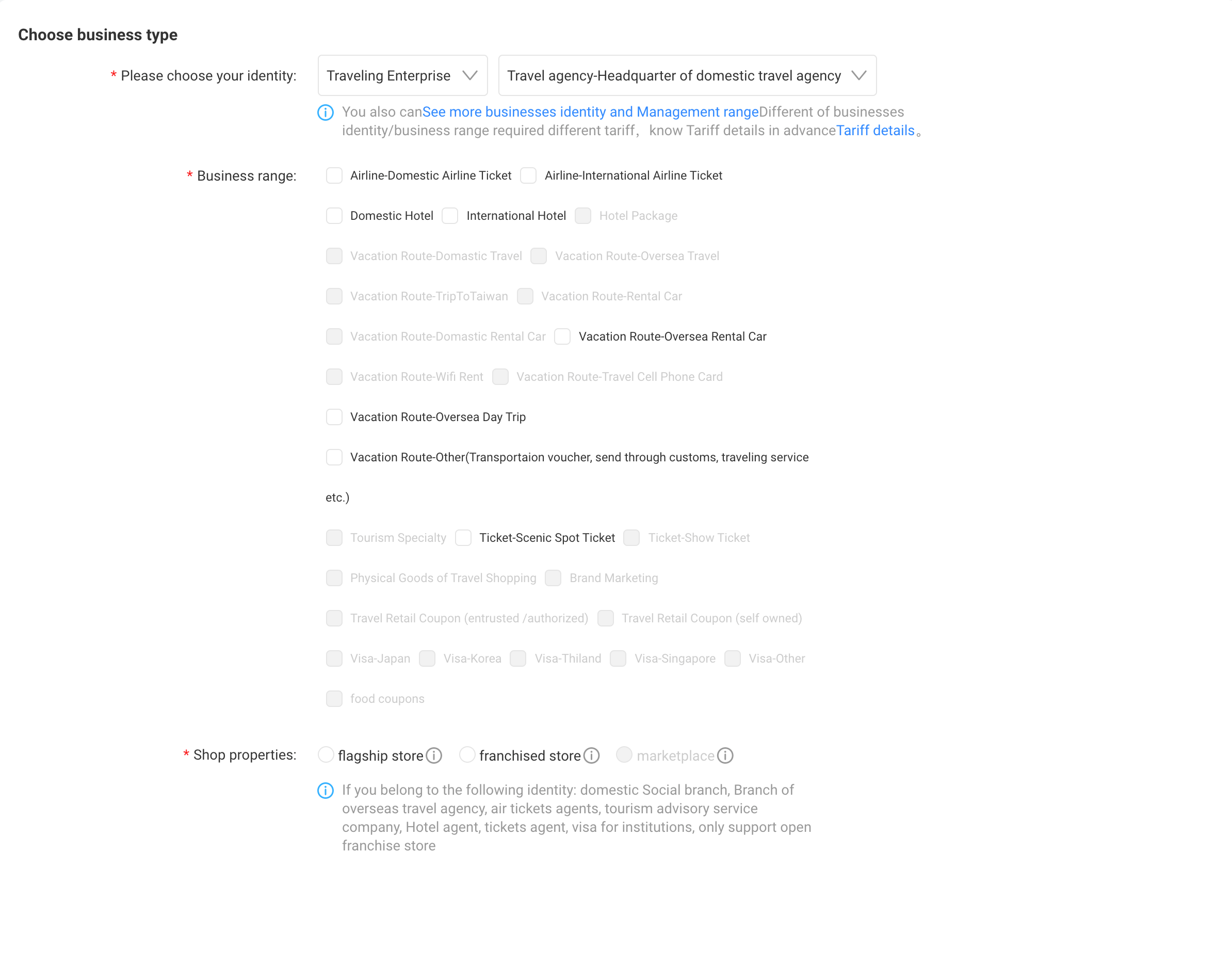This screenshot depicts an online form without a visible website interface, designed for selecting a business type. The form begins with a mandatory section titled "Choose Business Type" accompanied by red asterisks indicating required fields. 

The first mandatory field prompts users to "Please Choose Your Identity," with selectable options including Travel Enterprise, Travel Agency, and Headquarter. Additional information is provided below, indicating users can also select a "Business Identity" followed by a "Business Range," both marked with red asterisks to signify required input.

Options presented for "Business Range" include both selectable (in bold black) and non-selectable (grayed out) choices such as:
- Domestic Airline
- International Airline
- Domestic Hotel
- Vacation Route
- Overseas Day Trip
- Other Transportation Voucher
- Scenic Spot Ticket
- Rental Car

Further down, another mandatory field labeled "Shop Properties" requires choosing between:
- Flagship Store
- Franchise Store
With the "Marketplace" option grayed out and non-selectable.

Finally, the form specifies that only those belonging to certain identities (Domestic Social Branch or Branch of Overseas Agencies) can select particular options.